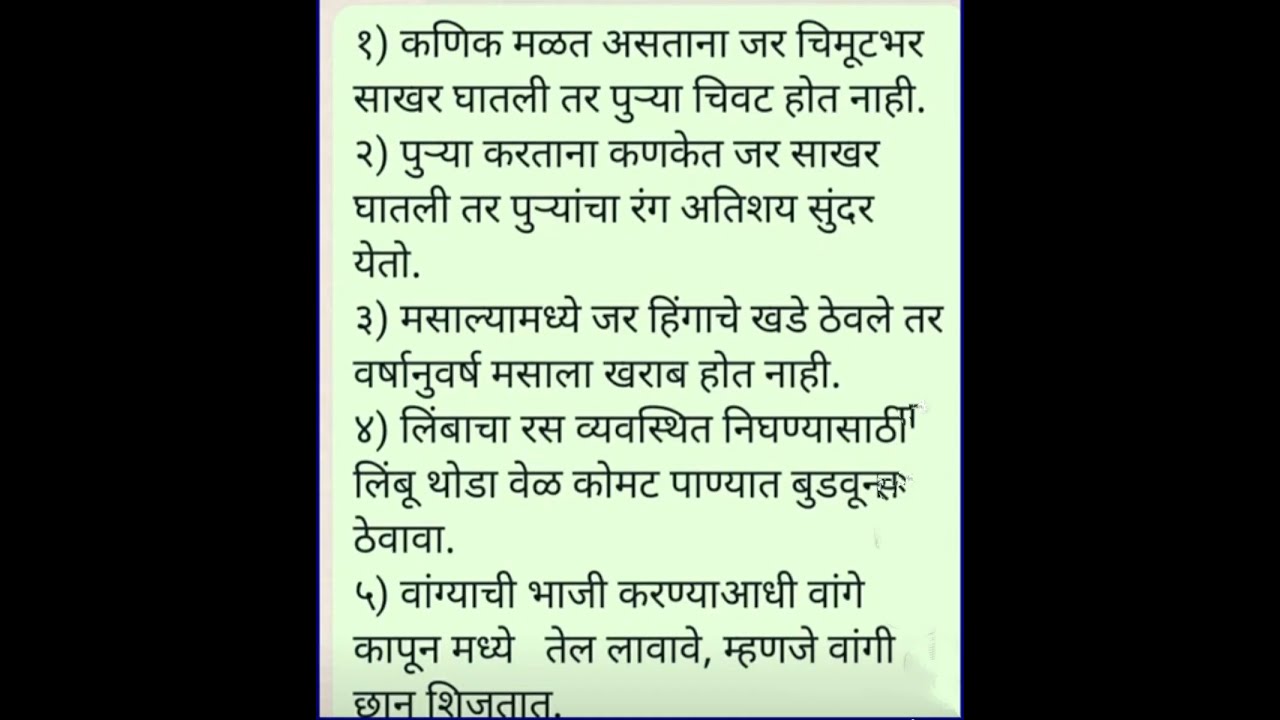The image features a central off-white piece of paper with black text in an Indian language, characterized by distinctive horizontal lines atop each letter. The paper contains three separate paragraphs formatted like a chat app screenshot, placed against a very light teal blue or grayish background. The entire composition is set within a widescreen frame, creating vertical black bars on both the left and right sides. The paragraphs of text are numbered sequentially from one through six, with gaps between each number, and are displayed in a consistent black font.